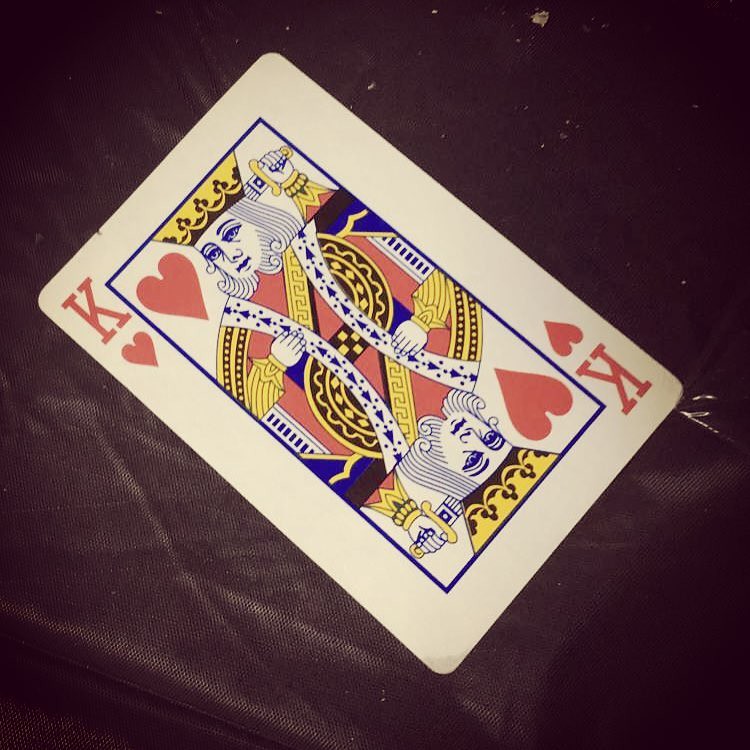This image features a detailed close-up of a playing card, specifically the King of Hearts. The card is prominently displayed on a table surface. The "K" and heart symbols are strikingly rendered in red. The king depicted on the card is adorned with a regal crown, colored in yellow and brown. His royal attire is a rich tapestry of blue, yellow, and red hues. Intriguingly, one of his hands holds a knife, positioned at the back of his head. The king also sports a distinguished white beard and mustache. The entire illustration is bordered by a blue outline, adding a touch of elegance to the card's intricate design.